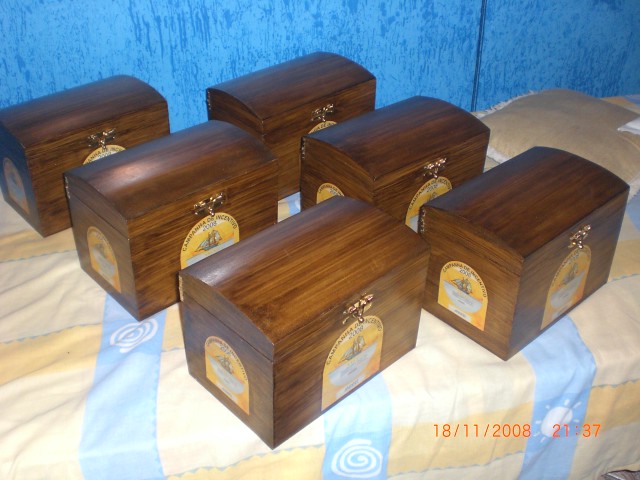This photograph captures a neatly arranged set of six small wooden storage chests placed on what appears to be a twin-sized bed, covered with a bedspread featuring a yellow and blue plaid design along with white spiral and sun patterns. These chests, distributed in two rows of three diagonal lines, each have a small golden metal latch for locking. Adorning each chest are indistinct yellow heart-shaped stickers featuring small white and black logos. The backdrop of the scene is a rough-textured, bright blue wall sprinkled with darker blue spots, adding depth to the setting. A tan throw pillow sits to the right of the chests on the bed. In the bottom corner of the photograph, faint text nearly blends into the background, reading “18-11-2008-2137,” which suggests the photo was taken on November 18, 2008, at 9:37 PM.